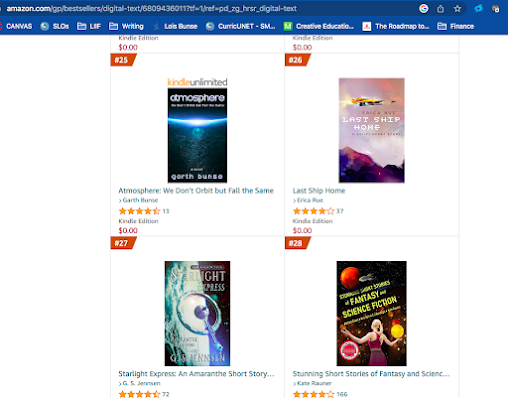The image depicts the Amazon.com bestsellers page in the Digital Text category. At the top, the URL reads, "Amazon.com bestsellers digital text." The web page header includes various text elements: "Canvas SMQs," "Writing," "Louise Owen," "Creative Education," "The Roadmap," and "Finance" on the top right.

The main section of the page showcases four digital texts:

1. **Top Left: "Atmosphere"**
   - **Title:** Atmosphere: We Don't Orbit, But Fall the Same
   - **Rating:** 4.5 stars (13 reviews)
   - **Format:** Kindle Edition
   - **Ranking:** #25
   - **Cover Description:** The cover features a space-themed illustration and includes the text "Kids Unlimited" and "Atmosphere."

2. **Top Right: "Last Ship Home"**
   - **Title:** Last Ship Home by Erika
   - **Rating:** 4 stars (37 reviews)
   - **Price:** $0.00
   - **Ranking:** #26
   - **Cover Description:** The cover depicts a spaceship and includes the title "Last Ship Home."

3. **Bottom Left: "Starlight Express"**
   - **Title:** Starlight Express: An Animation Short Story
   - **Rating:** 4.2 stars
   - **Ranking:** #27
   - **Cover Description:** The cover shows a spaceship and includes the title "Starlight Express."

4. **Bottom Right: "Stunning Short Stories of Fantasy and Science"**
   - **Title:** Stunning Short Stories of Fantasy and Science Fiction
   - **Rating:** 4 stars (166 reviews)
   - **Ranking:** #28
   - **Cover Description:** The cover features an image of a woman and the text "Fantasy and Science Fiction" written in yellow.

The background of the entire page is white.